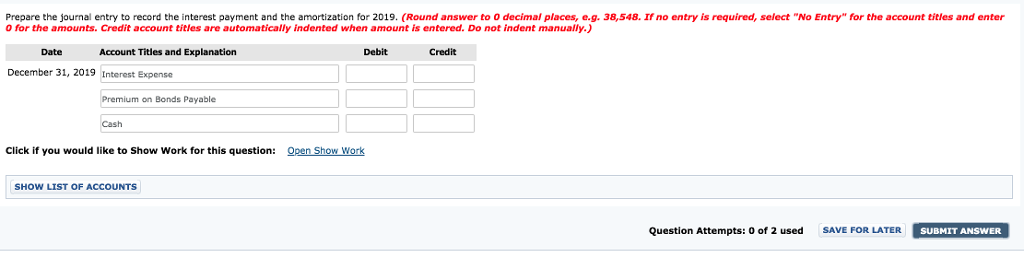The image shows a computer screen displaying a prompt for preparing a journal entry to record an interest payment and authorization for the year 2019. The prompt includes specific instructions to round the answer to zero decimal places and indicates that no entry is required if applicable, guiding users to select "No Entry" in such cases. Additionally, it notes that credit accounts will be automatically indented upon entry.

Below the instructions, there is a layout featuring three columns labeled: "Date," "Account Titles and Explanation," and "Debit" and "Credit." In the lower right-hand corner of the screen, there are two interactive buttons: "Submit Answer" and "Save for Later." This setup suggests that the screen could be part of either an accounting software or an accounting test, likely used in an educational setting such as a college course.